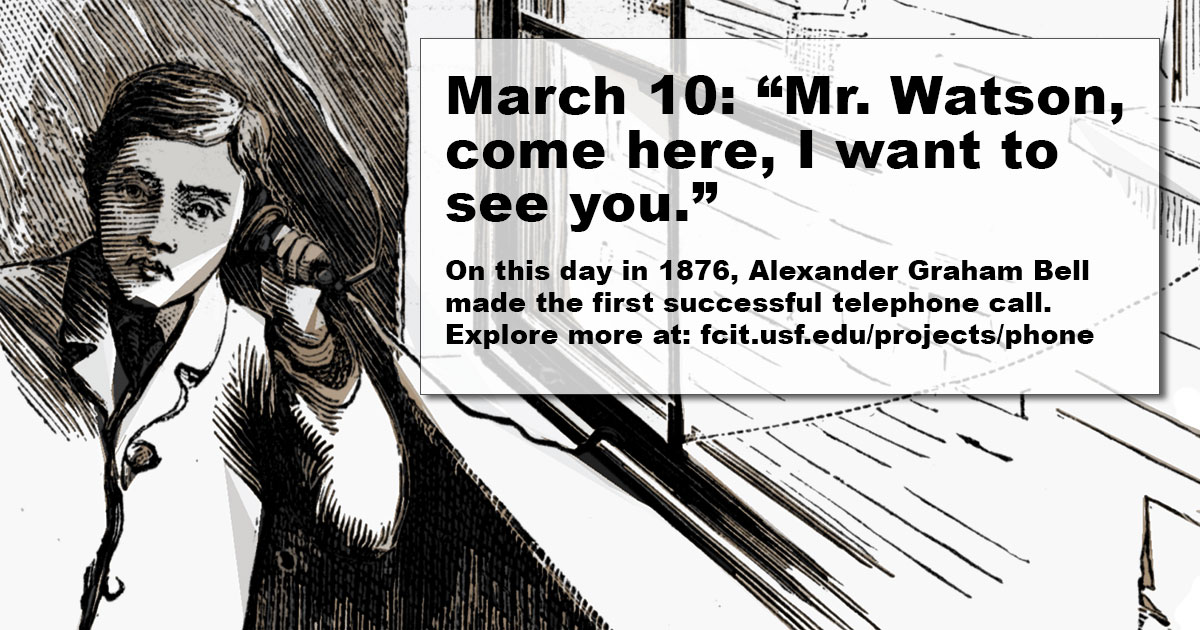This detailed black-and-white illustration, crafted in a hand-sketched or hand-drawn style, prominently displays a white background with black ink or sketching. At the center, a semi-transparent text box reads, "March 10: 'Mr. Watson, come here, I want to see you.'" Underneath, it notes, "On this day in 1876, Alexander Graham Bell made the first successful telephone call. Explore more at: fcit.usf.edu/projects/phone." On the left, a young boy with side-parted hair, dressed in a suit jacket, holds up an old-fashioned ear receiver next to a window, from which a telephone line extends. This historic scene vividly captures the moment of Bell's groundbreaking communication breakthrough.